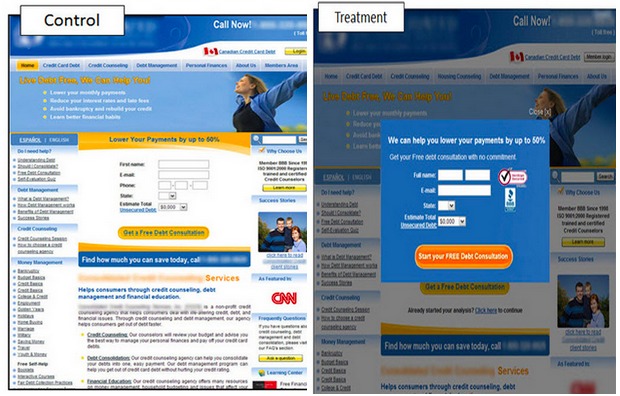The comparison includes two side-by-side images representing different websites, both aimed at offering debt consultation services. 

### Left Image: "Control" Website
- **Top Section**: The upper-left corner features a rectangle labeled "Control". At the top right, there's a prominent "Call Now" button.
- **Main Banner**: Dominating the top portion is a blue area showcasing a woman with her arms stretched out, suggesting relief or freedom.
- **Middle Section**: This area is dedicated to a sign-up form, asking for details such as Name, Email, Phone, and State. It includes a conspicuous "Get a Free Debt Consultation" button.
- **Advertisements**: The far right of the image is cluttered with advertisements, including a noticeable one for CNN.

### Right Image: "Treatment" Website
- **Top Section**: The top-left corner is labeled "Treatment".
- **Pop-Up**: Central to the page is a blue pop-up box. At the top, it claims, "We can help you lower your payments by up to 50 percent," and offers a "Free Debt Consultation with No Commitment". The form fields include Full Name, Email, State, and Estimate Total, followed by an orange "Start Your Free Debt Consultation" button.
- **Additional Elements**: To the right of the form, a black check mark is visible, alongside another box with a white background accented with blue. 

Overall, both images emphasize debt consolidation services, utilizing sign-up forms and bold calls to action to attract user engagement.